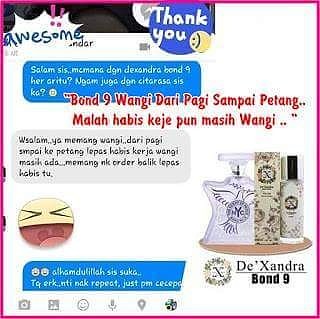The image is bordered with a thin pink line and primarily showcases a collage of text messages alongside decorative perfume bottles. On the left, the focus is on several text boxes filled with text in an unknown language, overlayed with dark red words that read: "Bondi, Wengi, Tari, Peji, Sem, Pei, Patang." Below this in red letters are additional words: "Mala, Habis, Kaji, Pon, Masi, Wagi." At the top, a blue circular icon with white lettering says "thank you" accompanied by a yellow smiley face emoji, and below it, the word "awesome" is written in green with purple exclamation points. A large, happy, smiling emoji sits below the text, adding a touch of whimsy. To the right of the image, there are several white perfume bottles with ornate decorations, each displayed on a round tan plate. The leftmost bottle features a dove, the middle bottle is tan, and the rightmost bottle is light gray. The lower right corner bears the text "D. Exandra" and "Bond 9" alongside an icon.